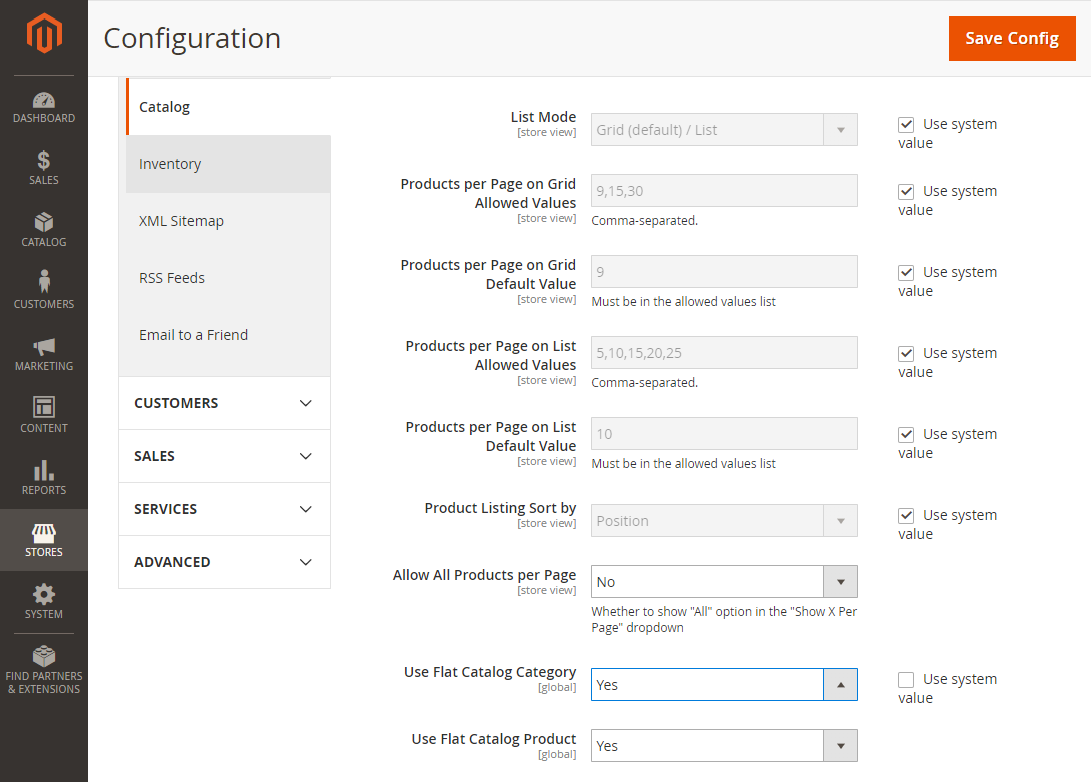This image is a screenshot of a computer screen displaying a configuration interface. At the top of the screen, the word "Configuration" is prominently displayed. The left panel has a dark background and features a vertical list of icons and labels. The icons, with the topmost one being orange, include options such as "Dashboard," "Sales," "Catalog," "Customer," "Marketing," "Content," "Stories," "System," and "Find Partners and Extensions."

To the immediate right of the sidebar, the interface is divided into four distinct columns. The first column lists categories like "Catalog" and "Inventory." The second column contains configuration settings such as "List Mode," "Products per Page on Grid," and "Products per Page on List," arranged in a vertical sequence.

The third column features fields for entering values, with some fields prompting for "Grid" input in a comma-separated format, "Must Be Allowed" values in a list, also comma-separated. Finally, the fourth column includes options for selecting existing system values, most of which are checked. At the top of this column is a prominent button labeled "Save Config."